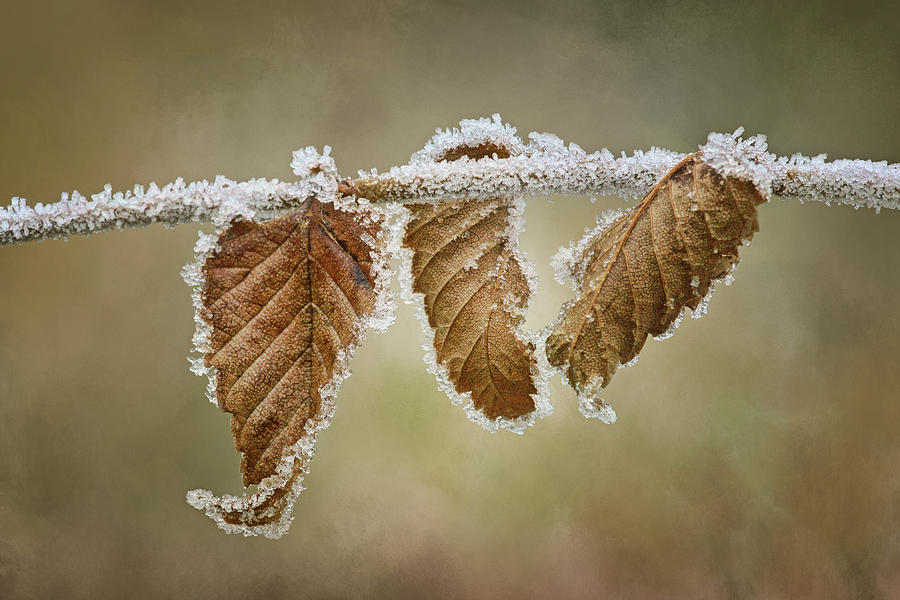An up-close, macro shot captures a thin branch extending horizontally from the left to the right side of the image, dividing it into one-third above and two-thirds below. The branch and its three dead, curled, and brown leaves are thinly coated with delicate frost, giving the appearance as if they were lightly salted. The largest leaf on the left hangs down in front of the branch, curving slightly at the end. The middle leaf, appearing partially torn, hangs behind the branch, while the smallest, slightly broken leaf on the right dangles in front. Frost outlines the edges of all the leaves and the branch, creating intricate ice crystal formations. The background features a soft, brownish blur with hints of olive green and gray, resembling a watercolor painting, adding depth to the wintry scene.